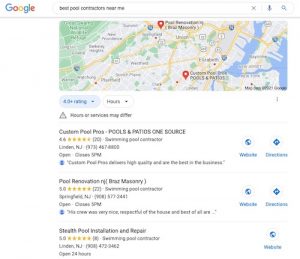The image is a computer screenshot featuring a Google search results page. At the top, there is a sleek, gray bar with rounded edges. On the left side of this bar, the Google logo is displayed in its signature colors. To its right, there is a search bar containing the text "Best Pool Contractors Near Me" in black lettering. The search bar includes a small gray 'X' on the far right. Adjacent to the search bar, there are typical Google icons for voice search and search submission: a microphone and a magnifying glass, respectively.

Below the gray bar, the screen shows a section of Google Maps with several red location pins indicating search results' locations. Directly beneath the map, there is a list of search results. The first result is "Custom Pool Pros," with a tagline "Pools and Patios One Source." Following that, the second result is "Pool Renovation," and the third is "Stealth Pool Installation and Repair." Each listing has a star rating, indicating customer reviews, along with their addresses and business hours. Notably, the first two results include buttons for visiting their website and getting directions, while the third listing only provides a directions button.

The image is relatively small, making finer details difficult to discern, and it becomes distorted when enlarged.